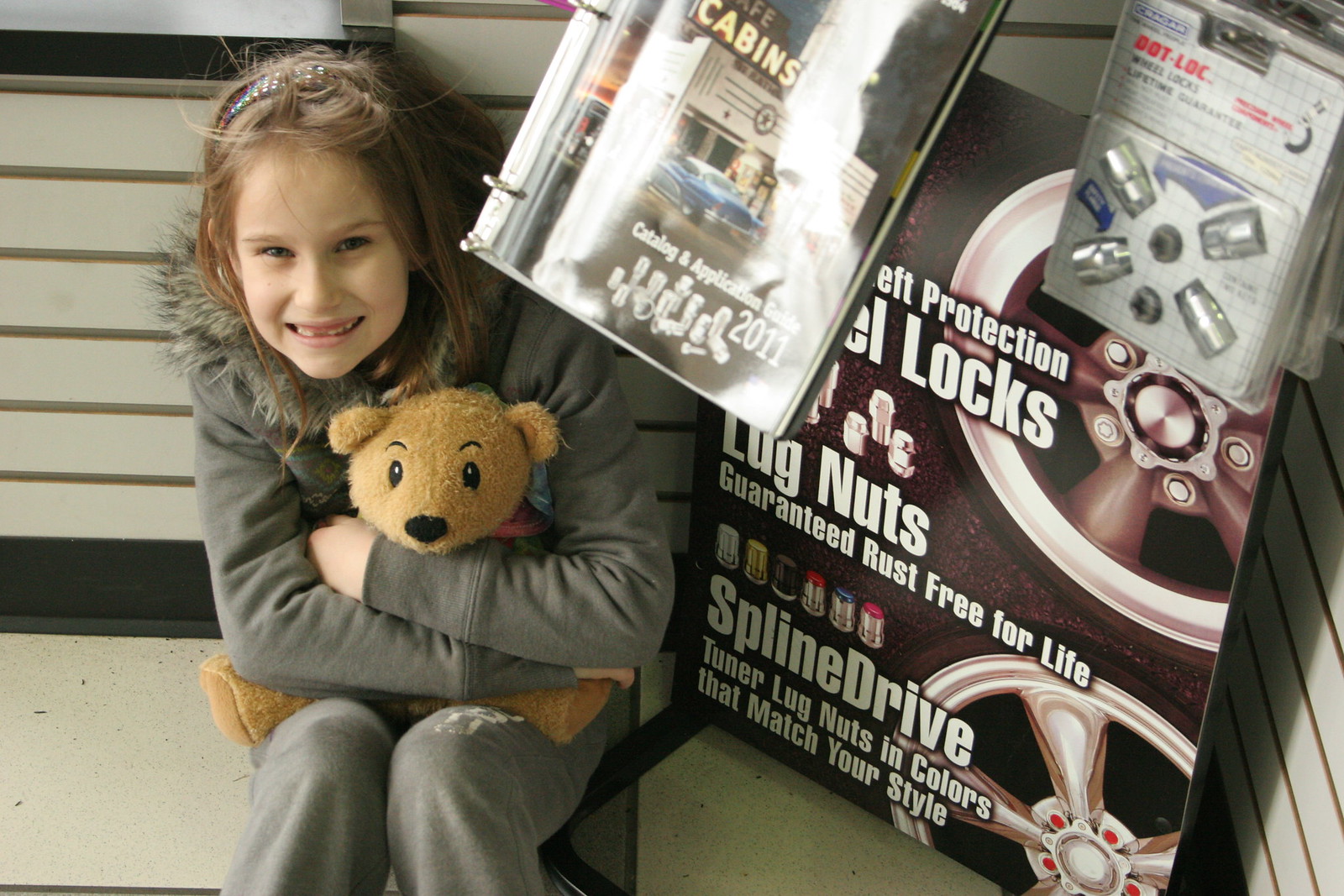In an indoor setting with white wooden walls and a tiled floor, a young girl with light brown, almost dirty blonde, hair sits on the floor in a gray hoodie with a fur lining and matching gray sweatpants. She holds a brown teddy bear close to her, her face arranged in a gentle, lip-parted smile. To her right in the corner of the room, there's a partially obscured automotive sign featuring images of tires and text about theft protection wheel locks and lug nuts, including phrases like "Guaranteed rust-free for life" and "Spline Drive tuner lug nuts in colors that match your style." A binder hangs in front of the sign, and an open book rests on a slender podium behind her.